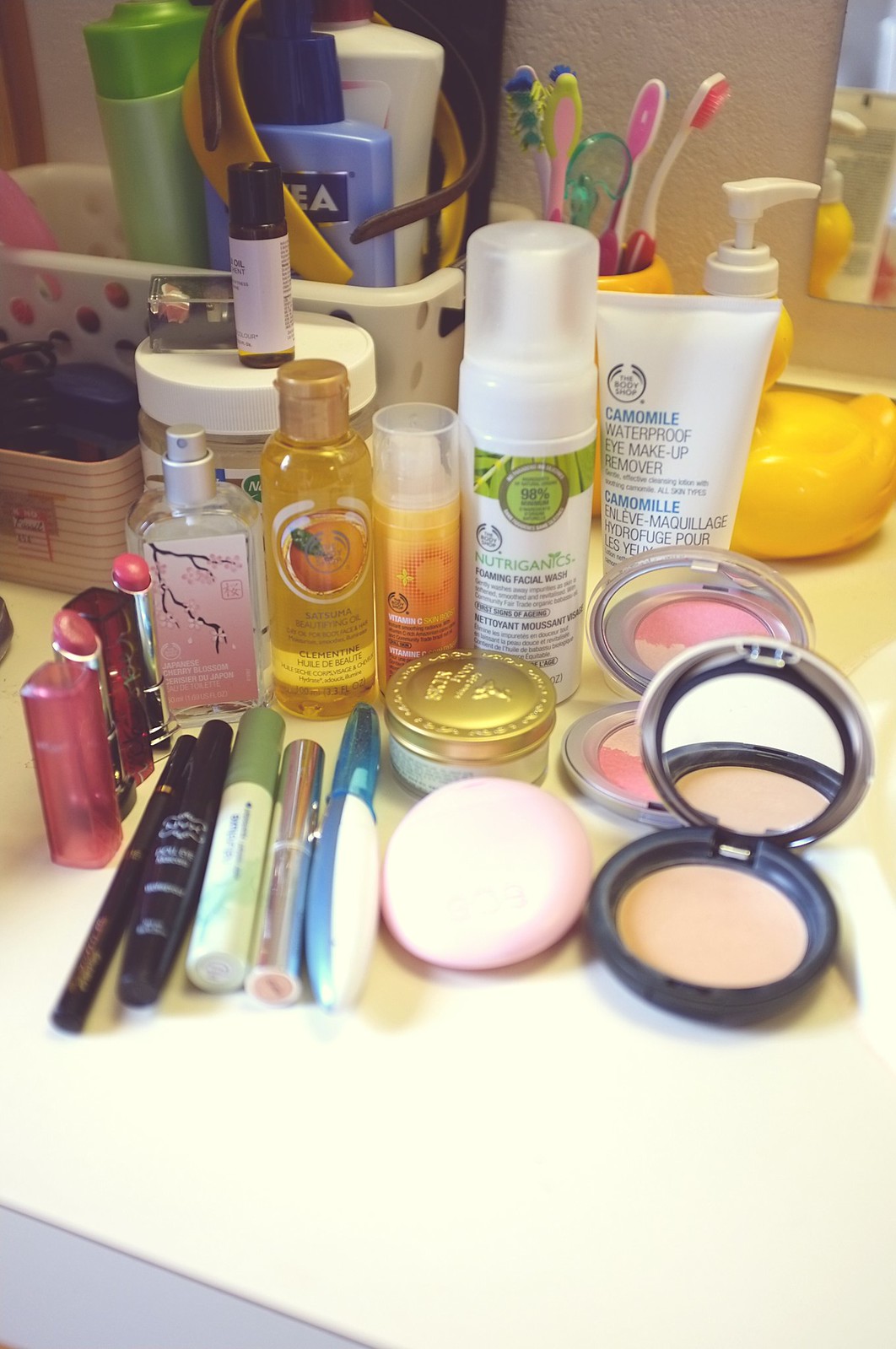This photograph showcases a cluttered bathroom countertop made of white Formica, featuring an assortment of beauty and personal care items. On the far right, just the lip of a sink is visible. Prominent on the countertop are various beauty products: a makeup sponge, powder, blush, multiple tubes of moisturizer, and a liquid hand soap dispenser. A cup holding several toothbrushes stands in the background, near a basket brimming with body lotions, over which a hairband is casually draped. Also visible in the background are a few perfume bottles and the tail end of a yellow rubber duck. In front of the body lotions basket sits a smaller basket containing unidentifiable black items. The countertop is densely packed, with lipsticks and eye makeup scattered amidst the other items. The background features a beige wall and the corner of a mirror positioned above the sink.